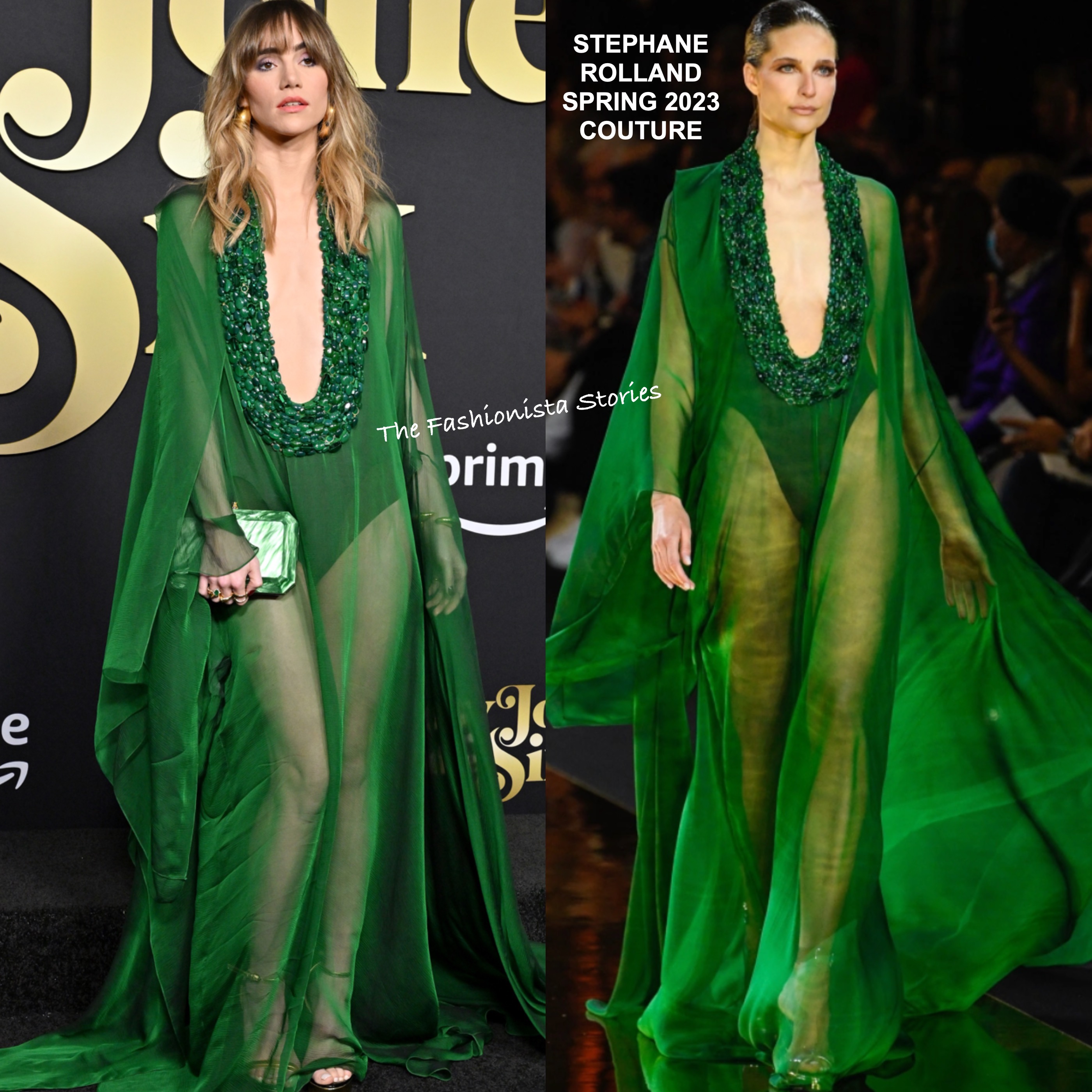The image is a magazine spread showcasing two women wearing identical designer gowns from Stéphane Rolland's Spring 2023 Couture collection. The gown is a striking green with see-through fabric on the arms and legs and a plunging neckline adorned with sequins or jewels that reaches near the belly button. It features long, flowing sleeves and a dark green cape draping elegantly to the floor. 

On the right side, a model with slicked-back hair struts down a runway, epitomizing high fashion. The text next to her reads "STÉPHANE ROLLAND, SPRING 2023 COUTURE" in all caps and white color.

On the left side, another woman with shoulder-length blond hair poses on what appears to be a red carpet. She carries a green clutch purse and wears a ring, her expression suggesting slight boredom or indifference. Between the two images, the text "The Fashionista Stories" is prominently displayed.